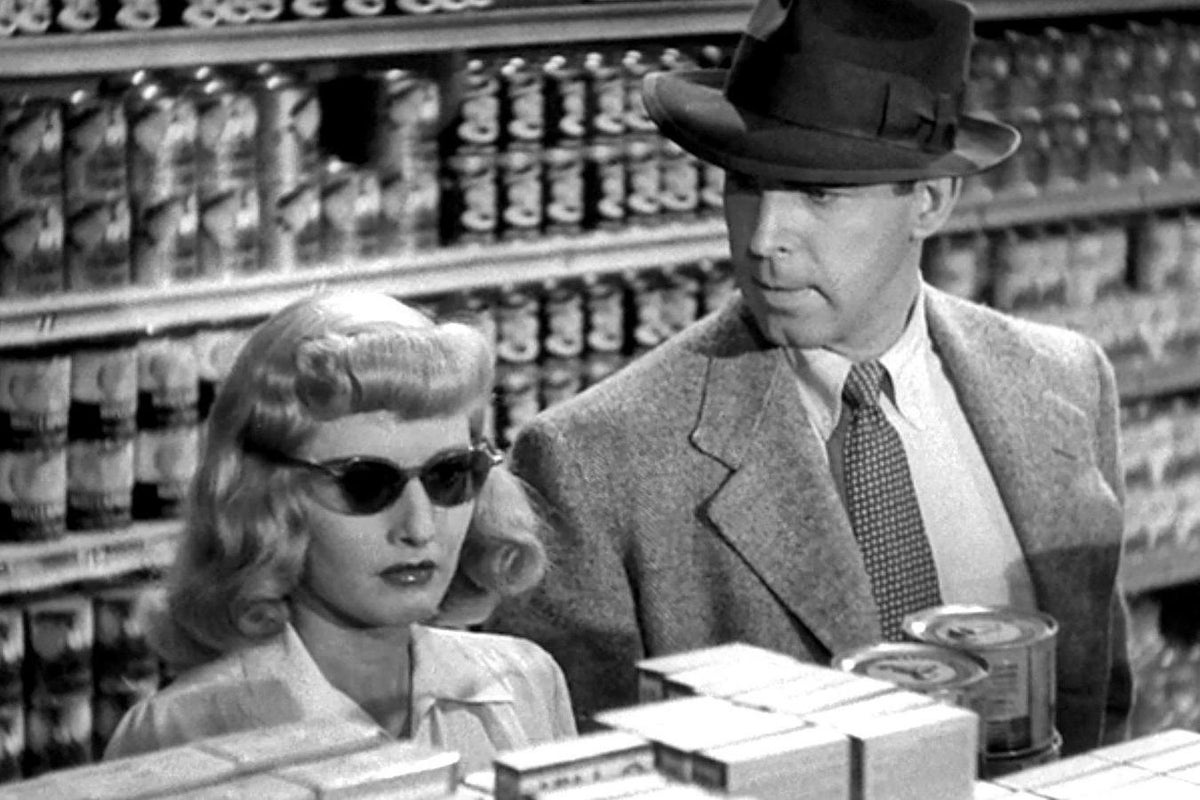The image is a still from an old black and white movie, likely from the 1950s, featuring Frederick Murray on the left and possibly Barbara Stanwyck on the right. They are standing in a grocery store, clearly indicated by the rows of canned goods visible in the background. Frederick Murray is dressed in a business suit and fedora, typical of the 40s and 50s era, and wears a serious expression, suggesting he might be warning the woman about something. The woman, shorter in stature, sports a pair of dark sunglasses often used to signify blindness in films of that period. She has a stylish, old-fashioned haircut with rolled-under bangs and bob, contributing to the film noir aesthetic. The scene captures a moment of tension or concern, with Murray intently staring at the woman as she looks ahead at the shelves, perfectly conveying the suspenseful vibe common in classic 50s cinema.